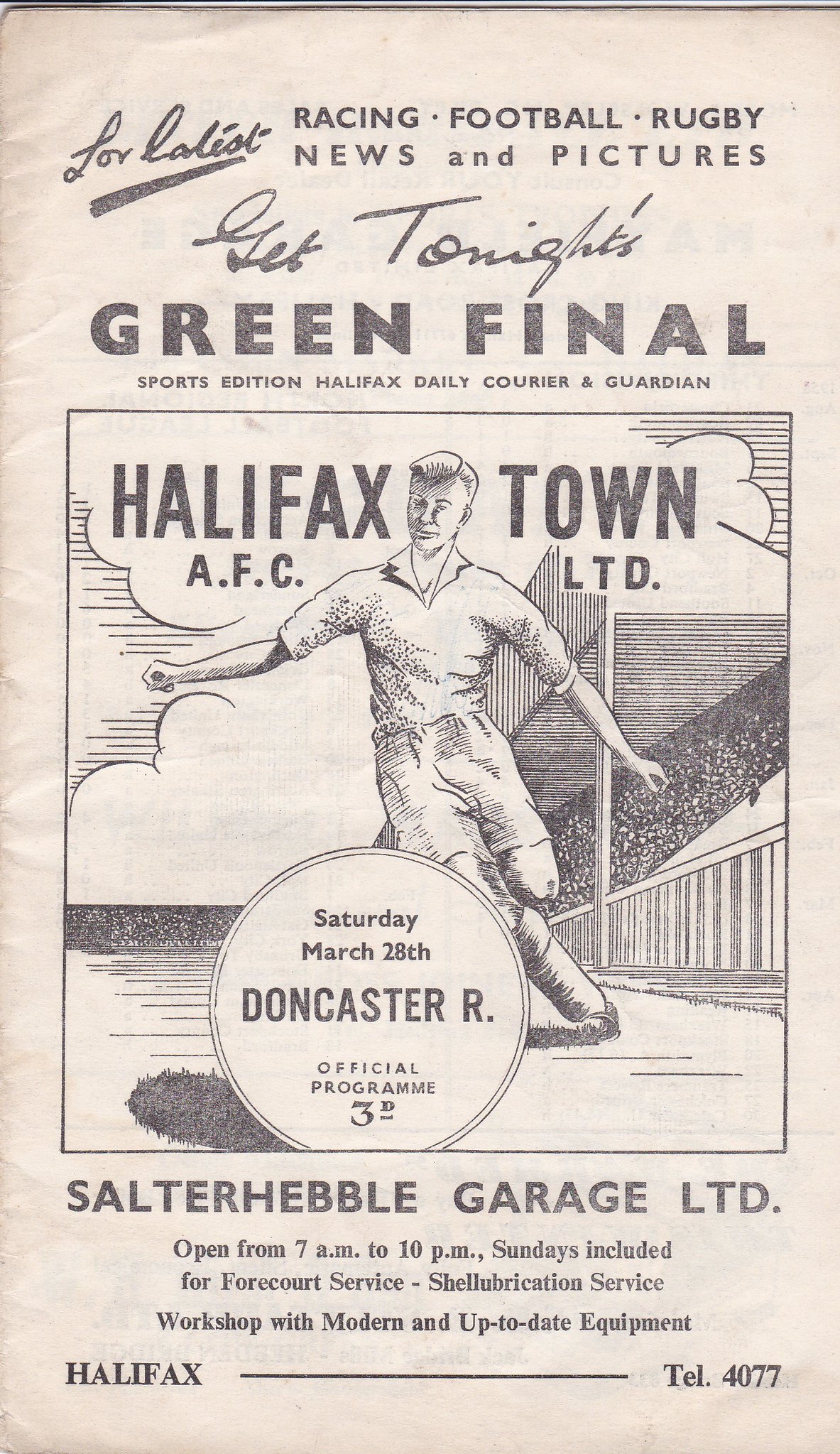### Detailed Caption:

This image depicts a tall, rectangular cover of an old sports program flyer, likely from the 1930s or 1940s. The paper is an off-white, light brownish color with noticeable creases along the left side, suggesting its age. The top of the flyer features bold black capital letters proclaiming "Racing Football Rugby News and Pictures," followed by a cursive text, "Get Tonight's Green Final." Beneath this, it reads "Sports Edition Halifax Daily Courier and Guardian."

At the center of the flyer, there's a square black-and-white illustration of a soccer player, rendered in a vintage style, possibly indicative of the 30s or 40s era. The soccer player is shown near the sidelines of a soccer field with a stadium on the right side. Above the player, a text overlaid on what appears to be a white cloud reads "Halifax Town AFC LTD." Positioned over the player's knee is a circular label stating "Saturday March 28th Don Caster Our Official Program 3D."

At the bottom of the flyer, it lists "Salter Hebel Garage Limited" with operational hours from "7 a.m. to 10 p.m. Sundays included," detailing services such as forecourt service and Shell lubrication. The garage boasts of "workshop with modern, up-to-date equipment." Closing the text, the flyer reads "Halifax" in capital letters, followed by the telephone number "4077."

This intriguing blend of advertisement and sports coverage encapsulates a bygone era, both in graphic style and commercial content, offering a nostalgic glimpse into the past.